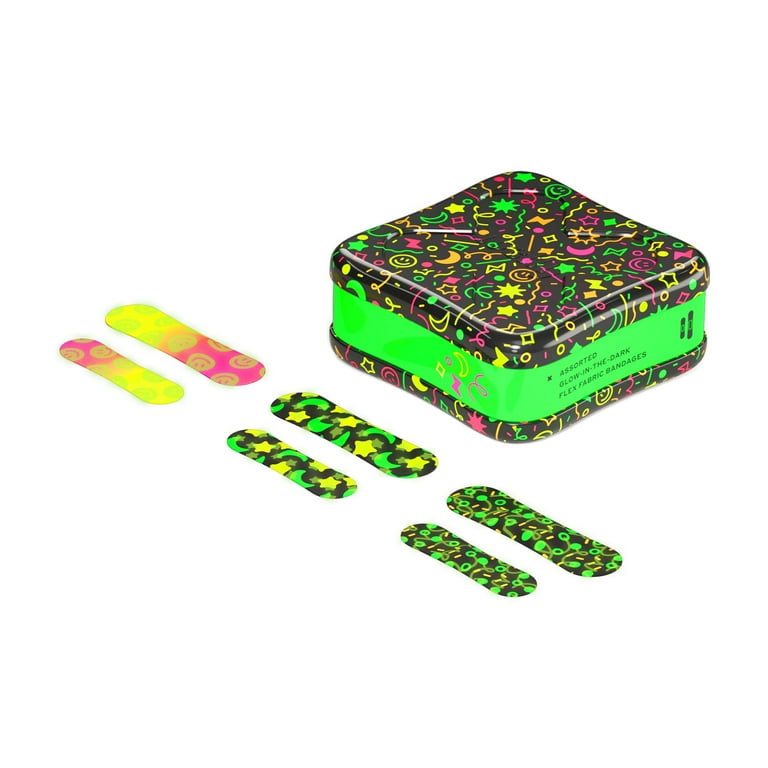The image showcases a vibrant and playful product: an assortment of colorful band-aids, displayed alongside their decorative case. The rectangular prism-shaped metal container features a striking design with a bright neon stripe wrapping around its center, while the top and bottom are adorned with a black background filled with multi-colored squiggles, smiley faces, green and yellow stars, orange and purple moons, and other festive symbols, creating a confetti-like appearance. The case also has a prominent green stripe along its sides, and the text "Assorted Glow-in-the-Dark Flex Fabric Bandages" is displayed. In front of the case, six bandages are neatly arranged in pairs, showcasing an array of sizes, colors, and patterns. Two bandages on the left are yellow and pink with playful smiley faces. The four bandages on the right are primarily neon green and yellow, featuring patterns such as moons and stars, as well as various shapes including circles, lines, and squiggles. This collection of band-aids, with its cheerful and eye-catching design, is perfect for adding a touch of fun to minor boo-boos.